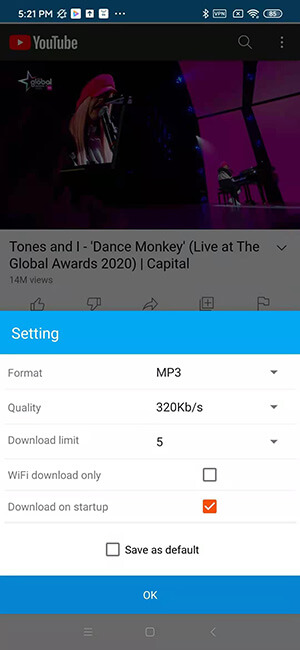This image is a screenshot of a YouTube video on a phone, captured at 5:21 PM. The top blue status bar displays the current time and various icons: an unclear stricken-through icon, the Google Play Store represented by a white square with a colorful triangle, an upward-pointing arrow, an ellipsis, an active Bluetooth icon, a WiFi symbol, and a battery indicator showing an 85% charge.

Beneath this, the YouTube interface is visible. The top banner is a red rectangle featuring a white arrow pointing right, and labeled "YouTube" in white text. To the right are a magnifying glass icon for search and a three-vertical-dots menu icon.

The screenshot captures a YouTube video paused on a scene featuring a woman with blonde hair wearing a pink hat and sitting in front of a piano with a microphone positioned close to her face. The background is vividly colored in a pink fuchsia hue. Another individual is visible in the background, also playing the piano.

Below the video frame, the video title is displayed: "Tones and I – Dance Monkey (Live at the Global Awards 2020)." Additional interface elements include a divider labeled "Capital" and settings options written in blue text. Indicated settings are: format as MP3, quality at 320 kilobytes per second, a download limit of 5, WiFi download only, and an active "download on startup" option highlighted in orange.